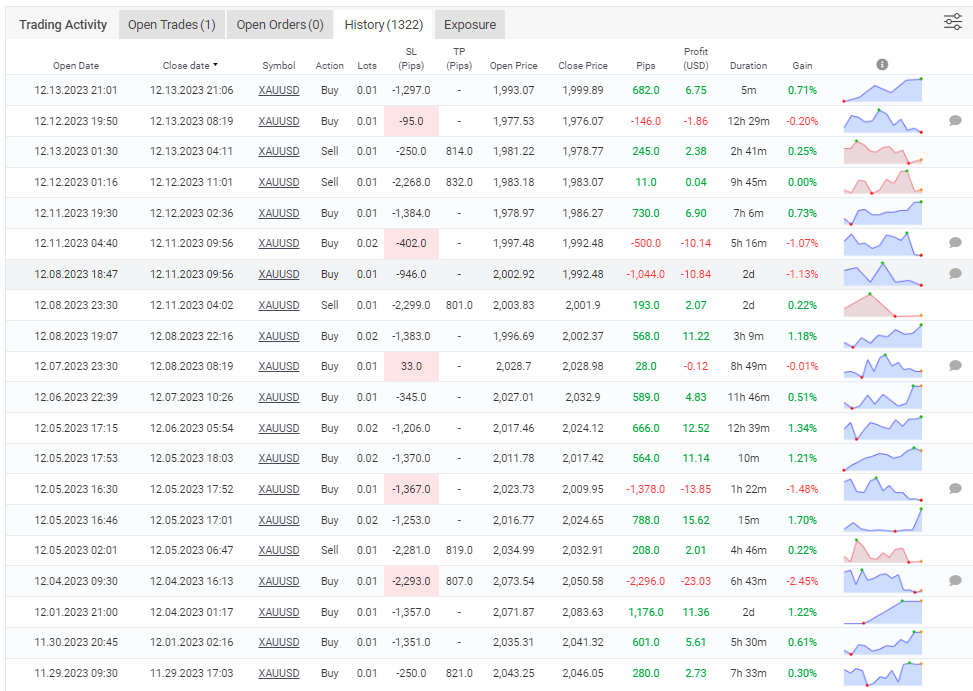The image depicts a detailed view of a data management system, likely resembling an Excel spreadsheet, specifically illustrating trading activities. At the top left, there are several tabs, with the active tab labeled "Trading Activity." Other visible tabs include "Open Orders (10)," "History (132)," and "Exposure."

Within the "Trading Activity" view, a table of data is presented. The table headers span across the top and include "Open Date," "Date Closed," "Symbol," "Action," "Lot," "SL (Stop Loss)," "TP (Take Profit)," "Open Price," "Closed Price," "Pips," "Profit (USD)," "Duration," and "Gain."

The first row of data contains the following details:
- Open Date: 12/13/2023 12:21:01
- Closed Date: 12/13/2023 12:21:06
- Symbol: XAU/USD
- Action: Buy
- Lot: 0.01
- SL (Stop Loss): -1,297.1
- TP (Take Profit): [Blank]
- Open Price: 1993.07
- Closed Price: 1999.08
- Pips: 682.0
- Profit (USD): 6.75
- Duration: 5 minutes
- Gain: 0.71%

Each trade is accompanied by a small chart, providing a quick visual reference for the trading activity. The data presented is thorough, showcasing key metrics important for evaluating the success and details of each trade within the period.